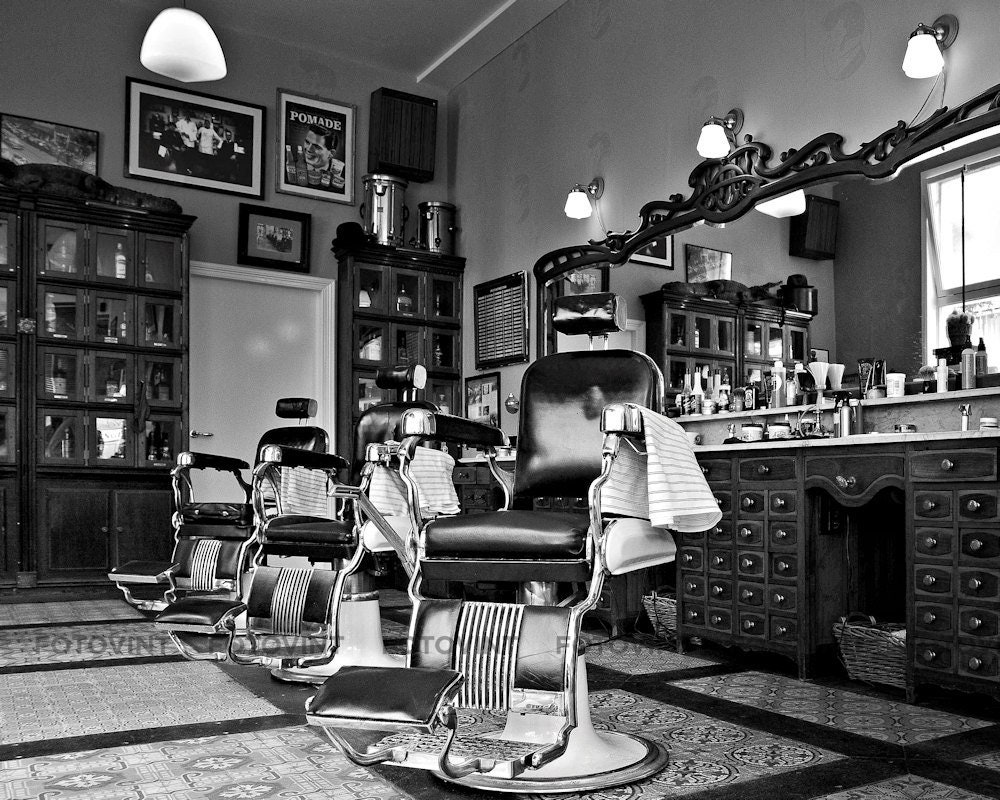This wide rectangular black-and-white photograph captures a meticulously maintained, old-fashioned barbershop, evocative of the 1920s or '30s. The tiled floor at the bottom of the image is notable for its intricate designs, where large squares are separated by thick black lines that guide the eye from the forefront to the rear left of the shop.

At the center, a prominent barber chair faces left diagonally. This chair, supported by a white circular swivel base, features black leather cushions on the armrests and seat, as well as metal footrests. Two additional chairs are placed behind it to the left, aligned in a row. Behind these, to the right, a large barber mirror with a black wooden frame reflects the shop's orderly arrangement.

The barbershop's interior is adorned with various pictures and posters, including one advertising pomade. Another poster showcases a group of barbers engaged in their craft. The shop is richly equipped with an array of barbering tools and products such as clippers, powders, and creams, which are neatly organized on the counter along with striped towels and a faucet. Numerous cabinets and drawers further denote a well-kept and high-maintenance establishment.

The ambient lighting, reminiscent of 1930s-style fixtures, illuminates the space under high ceilings, enhancing the shop’s classic aesthetic. With no people in sight, the three prominently displayed barber chairs—with their black cushions and metal leg rests—stand as the central features of this timeless, well-designed barbershop.